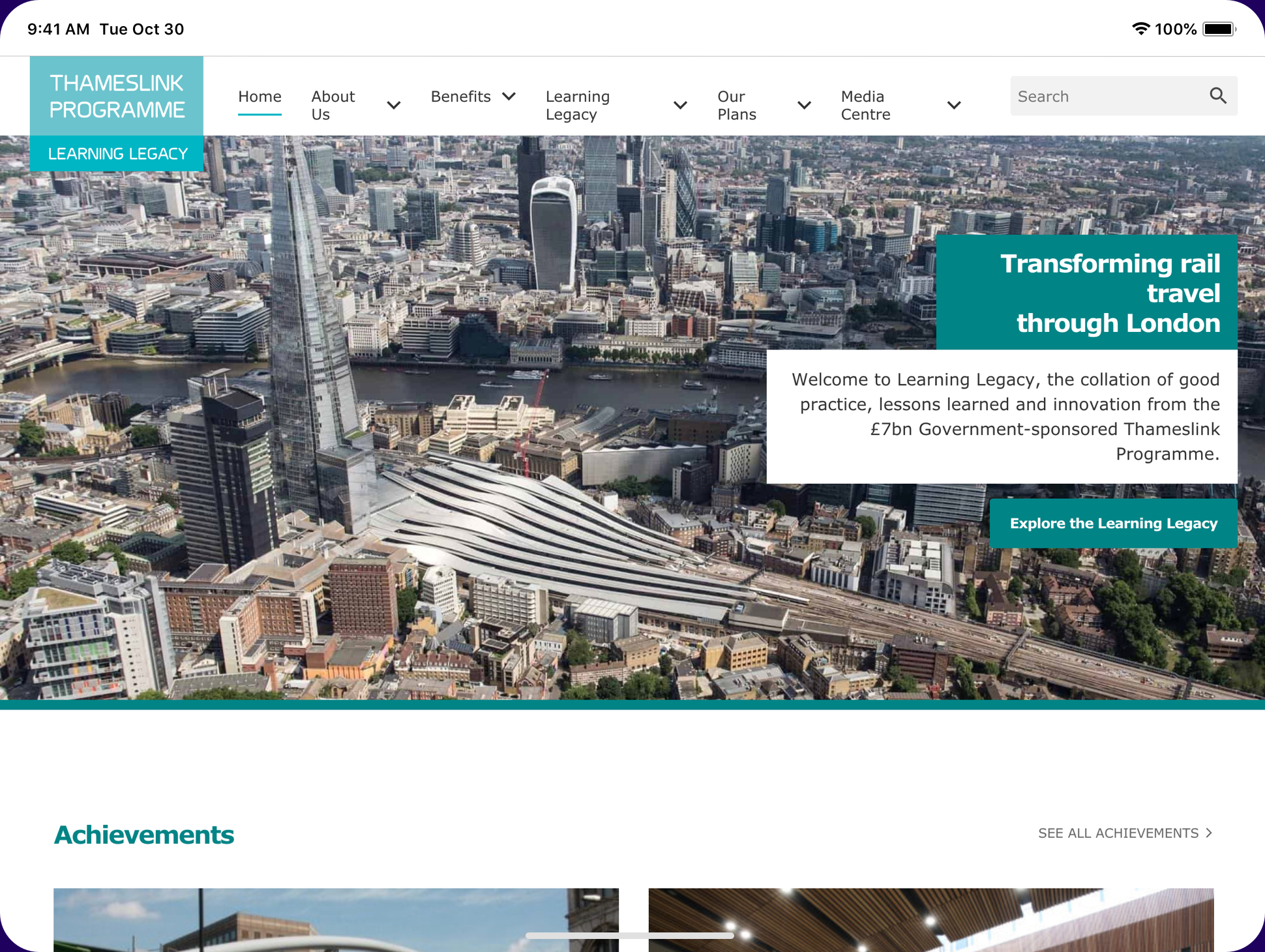The webpage appears to belong to the TEMSLINK program. In the upper right corner, there are icons indicating a full network connection and a fully charged battery. The upper left corner displays the time and date: "9:41 AM, Tuesday, October 30," in black text. Just below, there is a banner featuring the title "TEMSLINK Program" in white text on a sage green background. To the right of this banner is a navigation menu on a white background, listing options such as Home, About Us, Benefits, Learning Legacy, Our Plans, Media Center, and a search bar.

Central to the webpage is a large image of the Thames River flanked by a cityscape of skyscrapers and tall buildings, suggestive of a UK city. Prominently featured are a large train track and a mirrored skyscraper. Overlaid on the right side of this image is a green background with white text declaring, "Transforming Rail Travel Through London."

Beneath the image, the text welcomes visitors to the Learning Legacy, describing it as a coalition of best practices, lessons learned, and innovations from the 7 billion Euro, government-sponsored TEMSLINK program. An invitation to "Explore the Learning Legacy" follows.

Further down, in a white section, there is a heading that reads "Achievements" in green text. The image partially visible below showcases a blue sky and a ceiling structure, though details are indistinct.